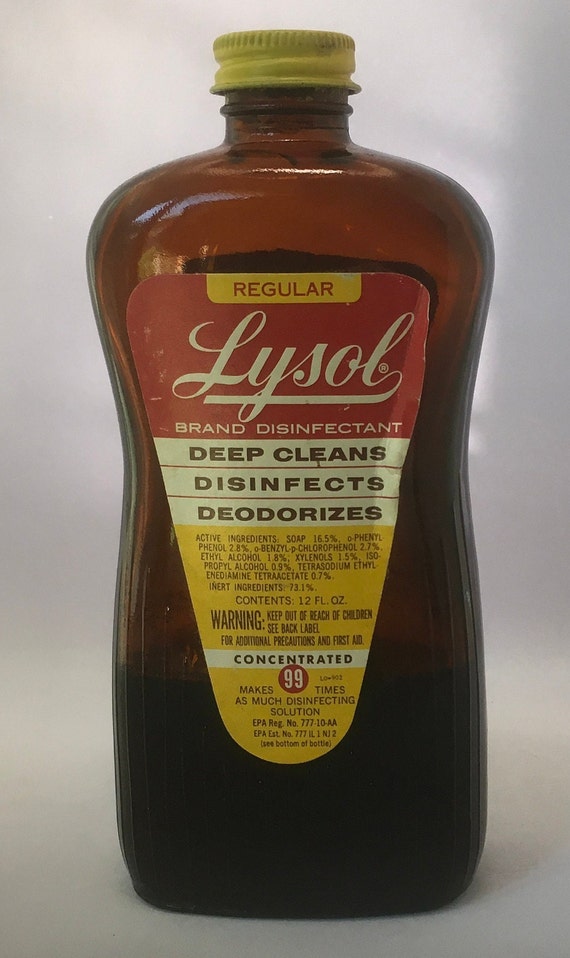The photograph is a vertically rectangular, full-color, and carefully staged image, created using artificial lighting. The background presents a gradient of gray shades, selectively illuminated by the light source, creating a soft backdrop without any borders. The focal point of the picture is an old glass bottle of Lysol, distinguished by its classic brown hue that transitions from a lighter brown at the top to a nearly black, tar-like shade at the bottom. This bottle is partially filled, with the liquid level reaching about a third of its capacity.

The bottle features a yellow metal turn cap, consistent with its vintage look. Prominently displayed at the front is an upside-down triangular label with rounded corners. At the top, a yellow bar holds the word “REGULAR” in red capital letters. Below this, the largest text on the label, “Lysol,” is inscribed in white cursive and underlined. Beneath it, in smaller capital letters, are the words “BRAND DISINFECTANT.” Following this are three distinct sections, each with white capital text set against a yellow background: “DEEP CLEANS,” “DISINFECTS,” and “DEODORIZES.” Toward the bottom of the label, additional information about the ingredients and a warning to keep out of reach of children appears in a smaller, more condensed text. Finally, there’s a white bar with the word “CONCENTRATED” and a red circle enclosing the number “99,” emphasizing the concentrated nature of the disinfectant. The combination of yellow, red, white, and black colors on the label stands out, providing a striking contrast to the neutral gray backdrop.